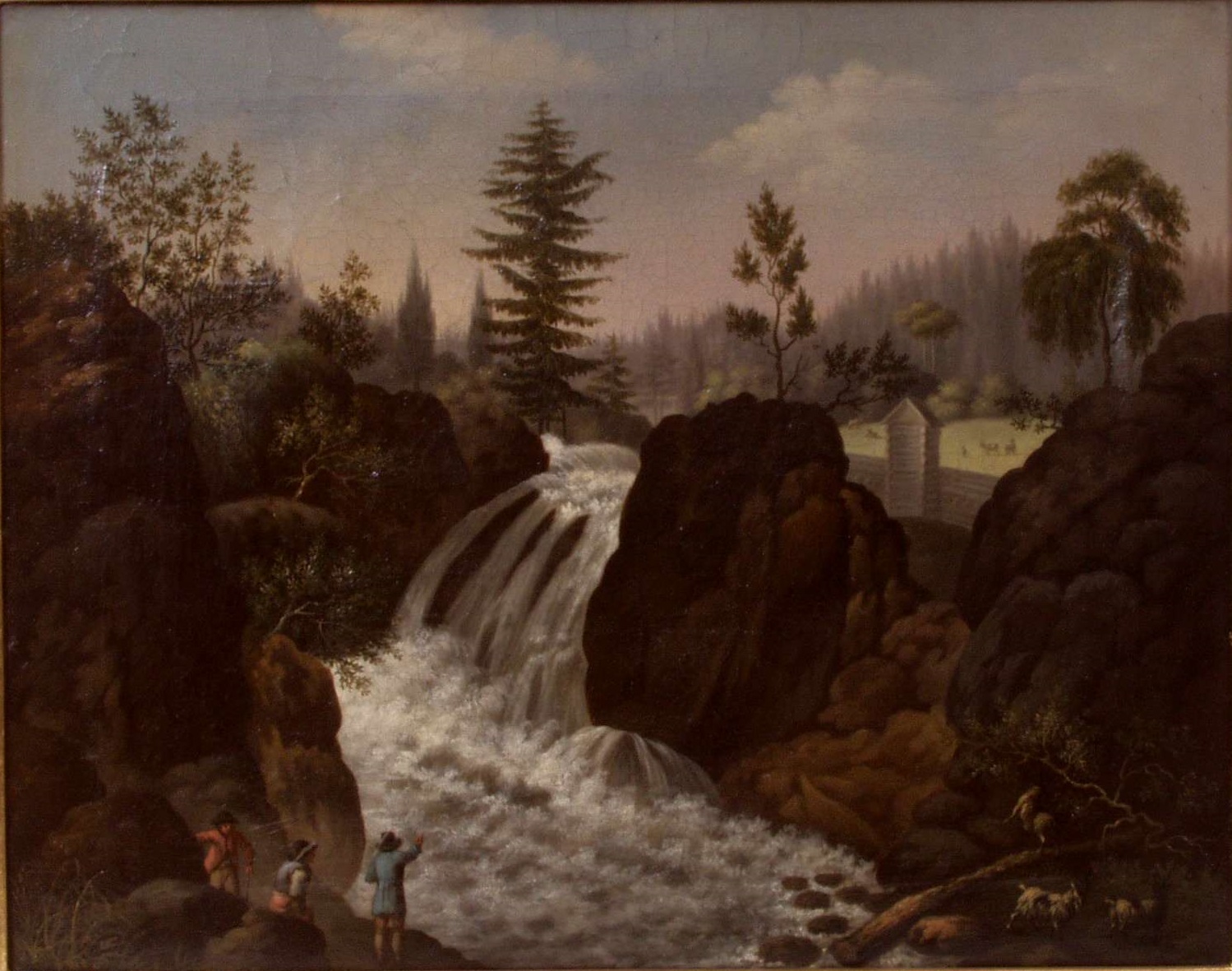In Christian August Lorenzen's dark, evocative painting titled "Helvetus Fossin," a dramatic waterfall cascades through rugged boulders into turbulent river rapids below. The painting, largely dark and somber in tone, captures the wild energy of the waterfall surrounded by large rocks and buttes. At the base of the waterfall on the left bank, three figures stand on smaller stones: one in a red jacket, another in a blue jacket, and a woman in a red and gray dress. On the opposite side of the riverbank, a lone individual with two goats stands atop a fallen tree. Central to the scene is a tall evergreen, seemingly sprouting from the waterfall itself. In the mid-ground, a narrow multi-story structure with a slanted roof can be seen nestled between two large boulders, resembling a small shelter or lighthouse. The backdrop reveals a dense forest of tall, narrow pine trees typical of a cold northern climate, fading into the distance under a sky painted with soft pinks, blues, and billowing white clouds. A guard tower and a tall wall appear to the right, augmenting the scenic yet perilous ambiance of the painting.